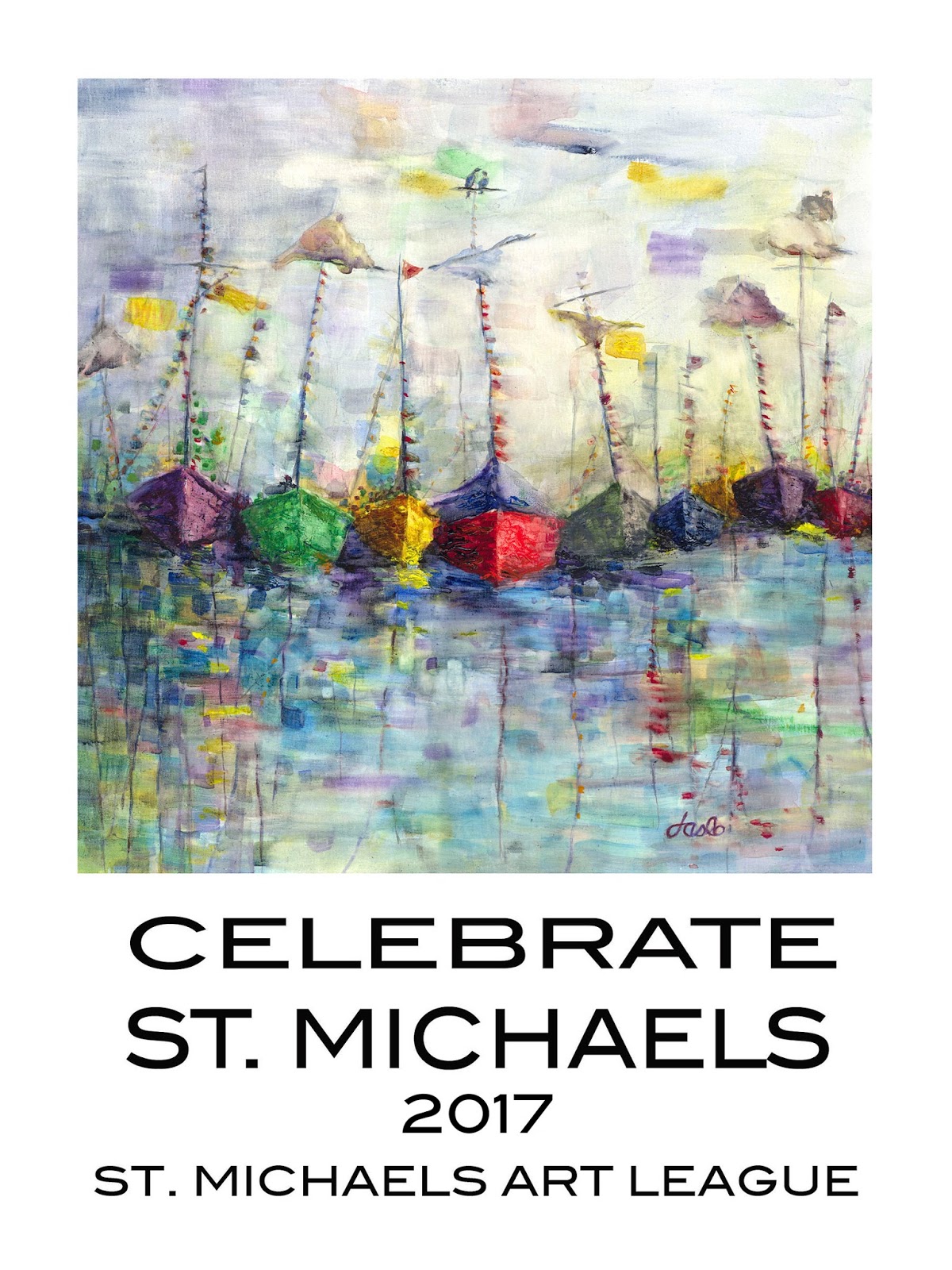The image is a vibrant painting that showcases eight boats aligned side by side on still water, viewed from the stern. The boats are distinctly colored in a sequence: brown, green, yellow, red, gray, navy bluish, deep brownish purple, and red. The water beneath them is a mesmerizing blend of yellow, blue, and purple brushstrokes, reflecting the boats in an almost abstract style. At the bottom of the painting, a small signature reads, "Celebrate St. Michael's 2017, St. Michael's Art League," indicating it was likely created for an event affiliated with the art league. Notably, two birds are perched atop one of the boats, adding a subtle detail to the colorful scene.